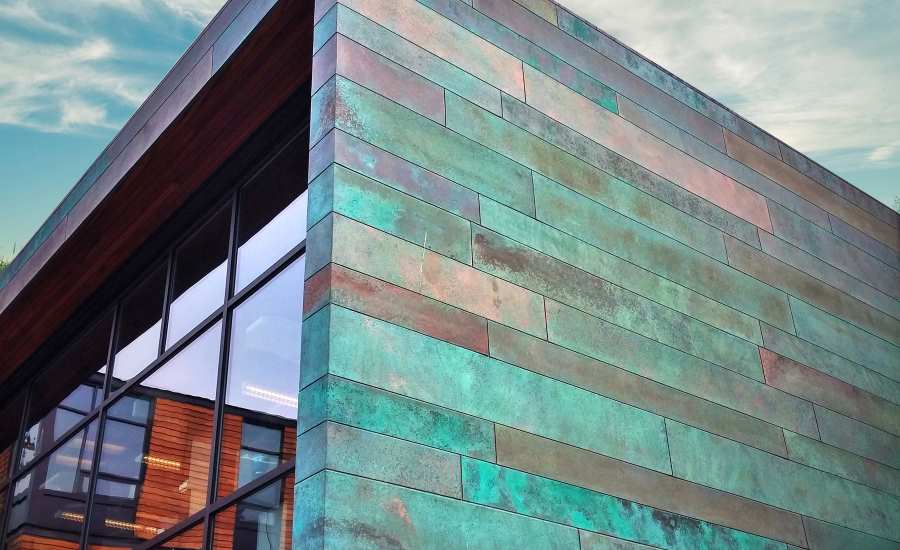This photograph, taken during the day from the ground looking up, features the side and partial front view of a striking modern building. The exterior is adorned with an array of metal blocks in varied sizes and a unique palette of colors—including aqua green, purples, blues, and hints of bronze, reminiscent of oxidized copper. The large, floor-to-ceiling windows with black aluminum frames on the left are highly reflective, showing the image of an adjacent structure clad in wood-like or brick-colored slats. The building's roof is visible in the upper left corner, where the sky, filled with wispy clouds and patches of blue, adds a serene backdrop. This highly artistic wall, possibly marking an office building, art gallery, or library, creates an intriguing visual with its grid of multicolored sections and the dynamic interplay of light and reflection.